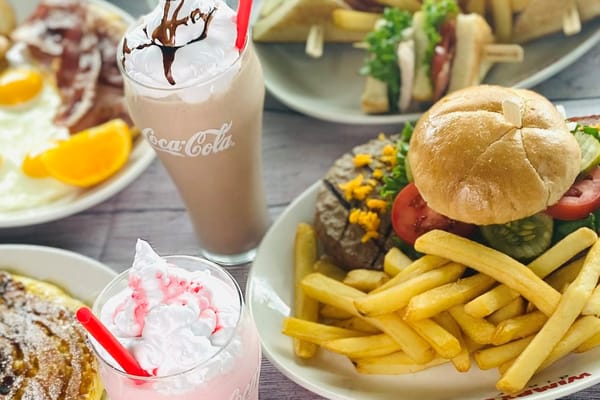The image captures a vibrant spread of dishes from a fast food restaurant or diner, probably for an advertisement or menu. At the forefront, there are two standout milkshakes: a Coca-Cola-themed malt milkshake in an iconic Coca-Cola glass, filled with light brown liquid, topped with whipped cream and hot fudge, and another pink strawberry milkshake adorned with whipped cream, pink syrup, and a red straw. Centrally placed on the table, a burger loaded with lettuce, tomato, onions, and pickles is accompanied by a heap of crisp, golden French fries. Adjacent to the burger, a club sandwich cut in half adds to the variety. In the background, other dishes can be seen, though they are slightly blurred; these include what looks like pancakes dusted with powdered sugar. The detailed and enticing presentation of these meals paints a clear picture of the diverse options available at this diner-style eatery.